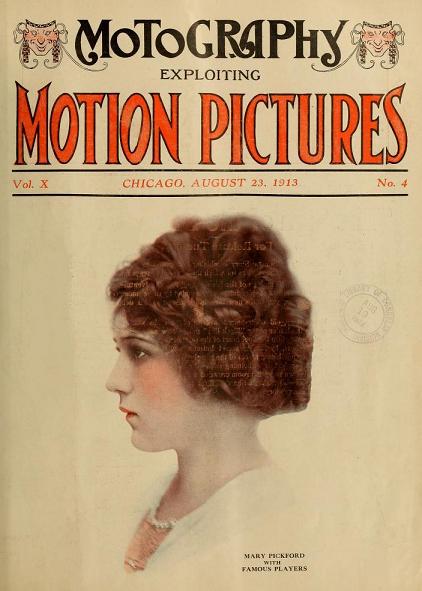This image features a vintage magazine cover titled "Motography," dated August 23, 1913, from Chicago. The cover prominently announces "Exploiting Motion Pictures" in bold red text and designates this as Volume X, Number 4. The magazine aims to educate readers about the burgeoning world of motion pictures, a novel and revolutionary medium at the time. Centered on the cover is a profile image of Mary Pickford, a celebrated actress of the era, donning a white dress and a necklace, accompanied by the mention of her association with Famous Players. The text is displayed in classic old-fashioned print, with notable sections highlighted in alternating red and black text, enhancing the vintage aesthetic of the publication.